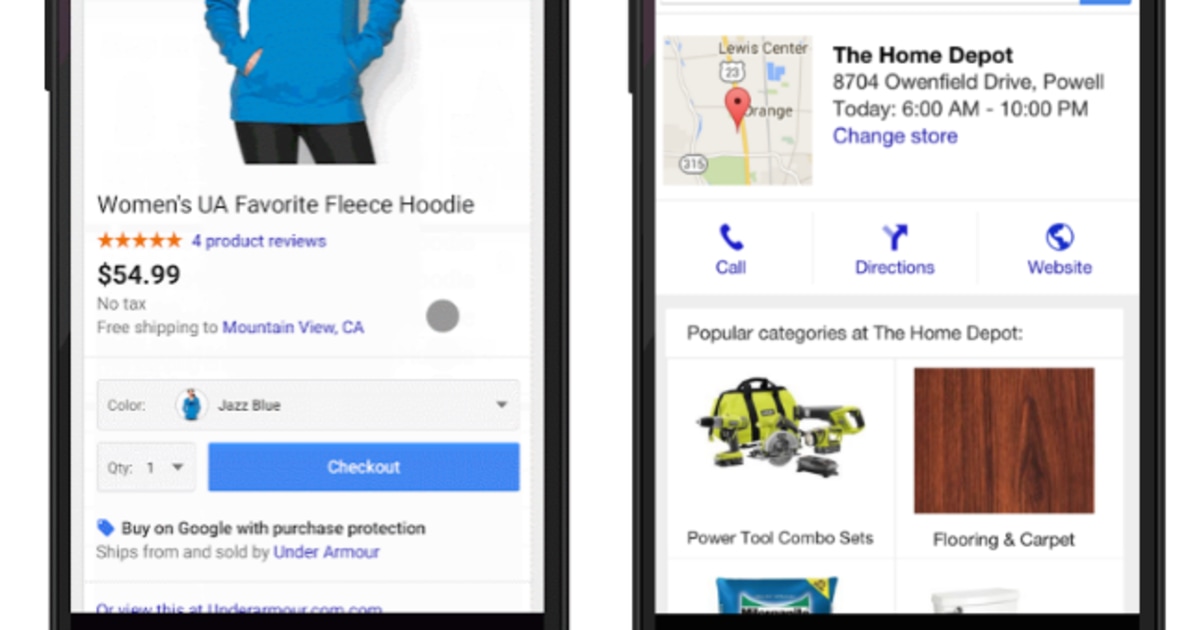In the image, there are two distinct screenshots taken from cell phones, displayed side-by-side. The left screenshot showcases a product listing for a woman's fleece hoodie. The hoodie, modeled by a figure whose upper body is not visible, is a vibrant blue color, referred to as "jazz blue." The model wears the hoodie paired with black pants. This fleece is priced at $54.99, with an option for free shipping from Mountain View, California. The interface includes a large rectangular checkout button prominently featured.

The right screenshot displays details about a Home Depot store. It includes a small map, the store's address, and current operating hours, which today are from 6 a.m. to 10 p.m. Additionally, there are three interactive options that allow the user to call the store, get directions, or view the website.